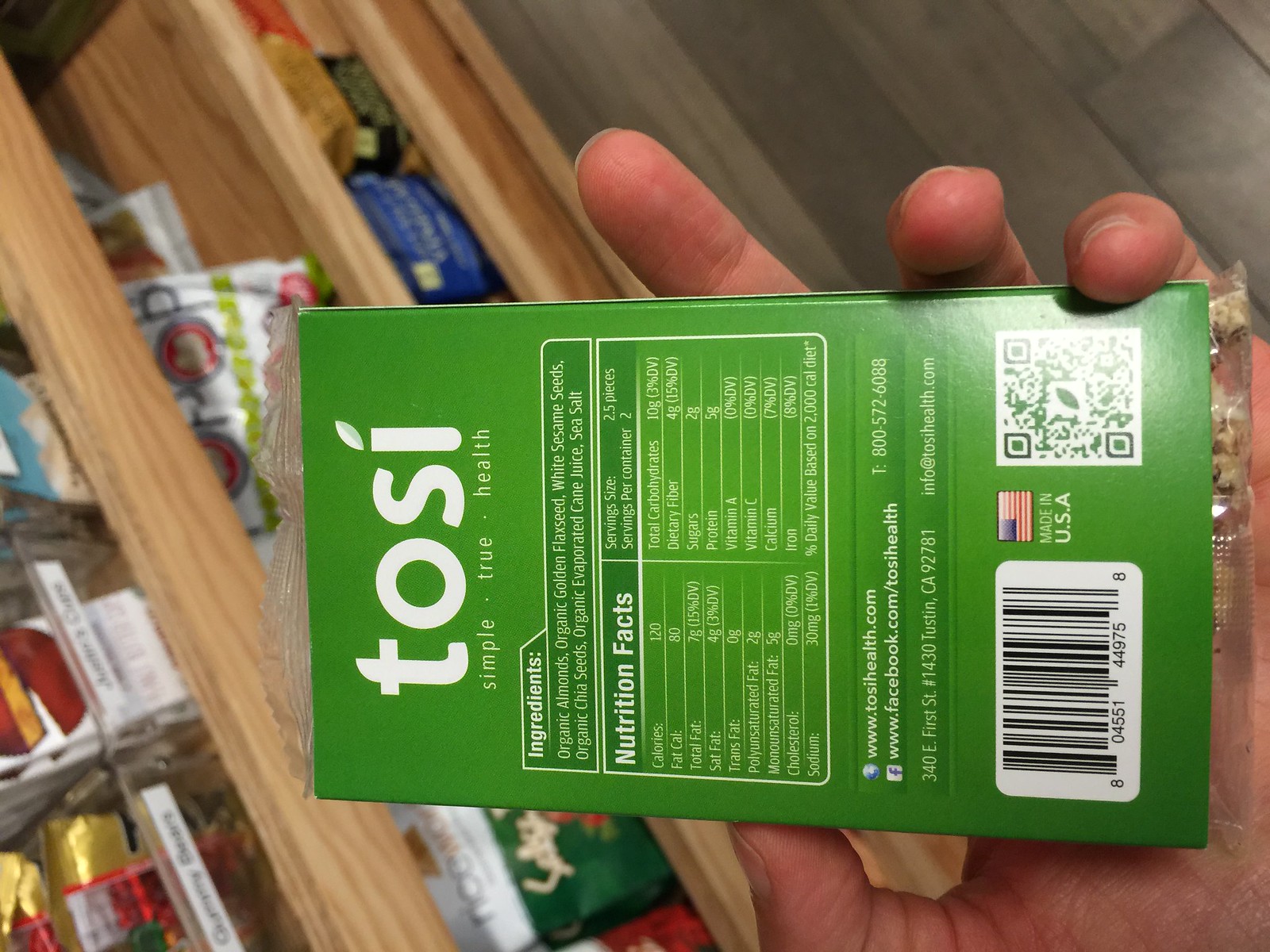The image showcases a green box with its text oriented horizontally, making it challenging to read. At the top of the box, "Tosi" is prominently displayed in white text, where the 'i' is creatively replaced with a small leaf symbol. Below this brand name, the phrase "Simple. True. Health." is written, emphasizing the natural and healthy nature of the product.

The ingredient list includes "organic almonds," "organic golden flaxseed," "white sesame seeds," and other wholesome components. The box also features nutrition facts, though they are partially obscured and difficult to decipher. Additionally, the packaging provides the website "TosiHealth.com" and a Facebook link for further information. A UPC label, a QR code, and an American flag icon indicating "Made in USA" are also visible on the box.

A left hand holds the box, with a background that includes shelves on the left side displaying various products such as chips and chocolates. The ground features a dark brown laminate flooring, adding a warm, rustic touch to the scene.